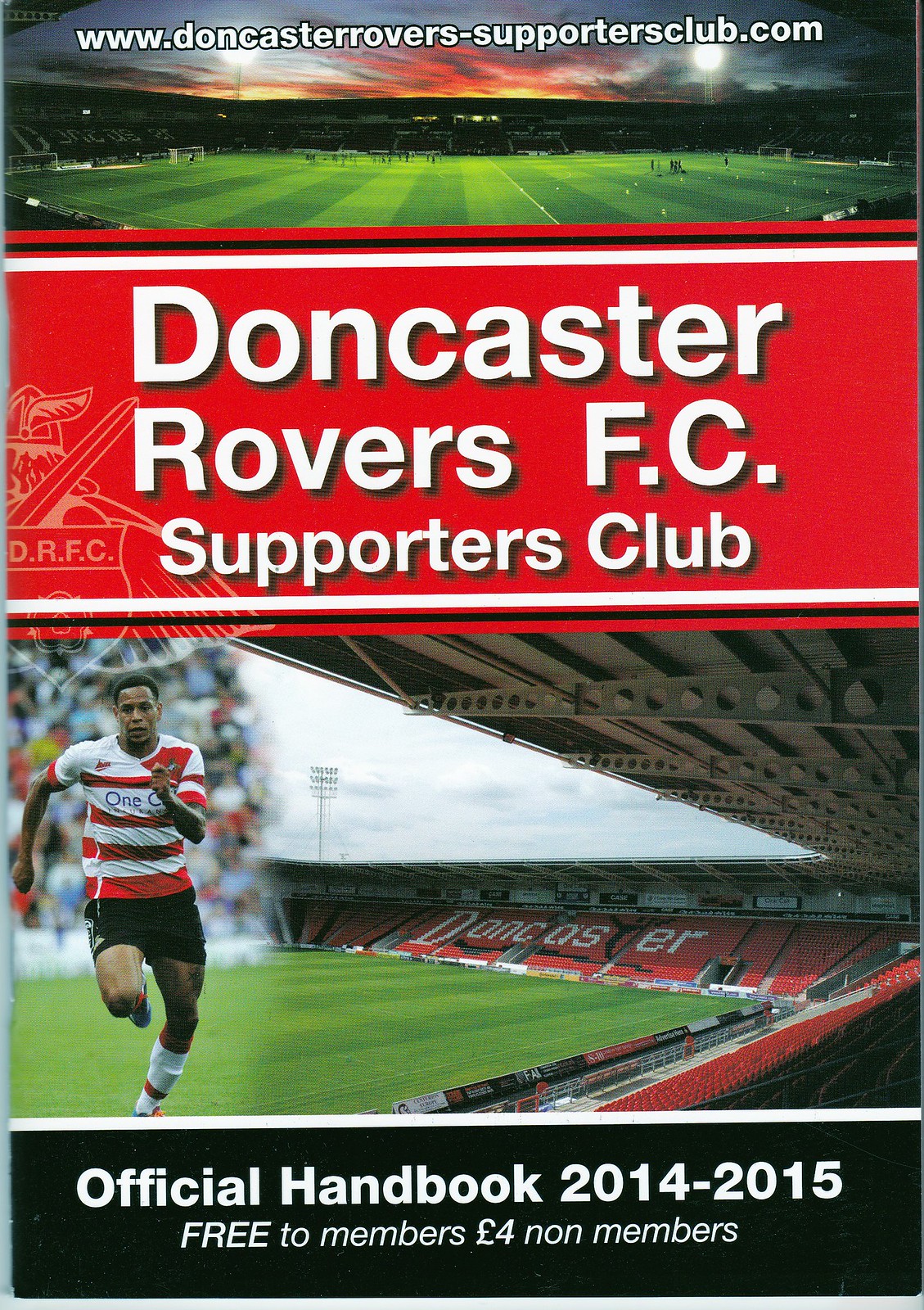This poster advertises the Doncaster Rovers FC Supporters Club and features detailed visual elements. At the very top, in white text, the website www.doncasterrovers-supportersclub.com is displayed. Below this, a full-scale landscape photo showcases a green striped soccer field surrounded by stands. Underneath, a thick red background with black and white stripes hosts the inscription "Doncaster Rovers FC Supporters Club" in white text. On the left side of this section, there is a grey illustration of the team's badge, depicting a knight with a sword over his shoulder, wearing a helmet and cape, and holding a shield with the letters "DRFC" and a small flower beneath it.

Beneath this section, another photograph captures the stadium from an angle, focusing on the narrow end of the field. The seats, all red, spell out "Doncaster" in white text, with the "T" being black. Below this photo, a thin black strip contains white text that reads "Official Handbook 2014-2015 Free to Members for British Pounds Non-Members." Additionally, there is an image of a soccer player running on the left side, enhancing the dynamic and vibrant feel of the poster.